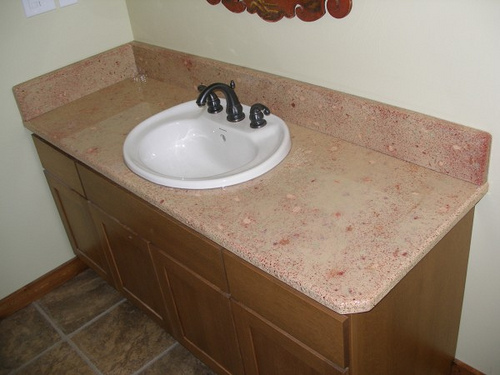The image showcases a bathroom countertop seamlessly integrated into a corner where the longer side abuts the right wall and the shorter side touches the left wall. The countertop is made of smooth, rose pink granite and features a centrally-placed white sink with a black metal faucet and accompanying fixtures. Above the countertop, on the wall, is the bottom portion of a swirly wooden frame, presumably for a mirror or another form of wall décor.

The luxurious countertop is supported by brown wooden cabinetry. The cabinetry includes two central doors and possibly additional doors on either side, designed without visible handles, suggesting they either slide open or can be grasped along edge crevices. Above the cabinet doors are three drawers: a very wide one in the center and two narrower ones on either side. Notably, the two side drawers are slightly ajar, confirming their function as storage compartments. 

The floor below is adorned with light and dark brown marble tiles, arranged in a square pattern. The flooring is complemented by brown wood borders, adding a touch of elegance to the overall aesthetic of the bathroom space. The image does not contain any text.